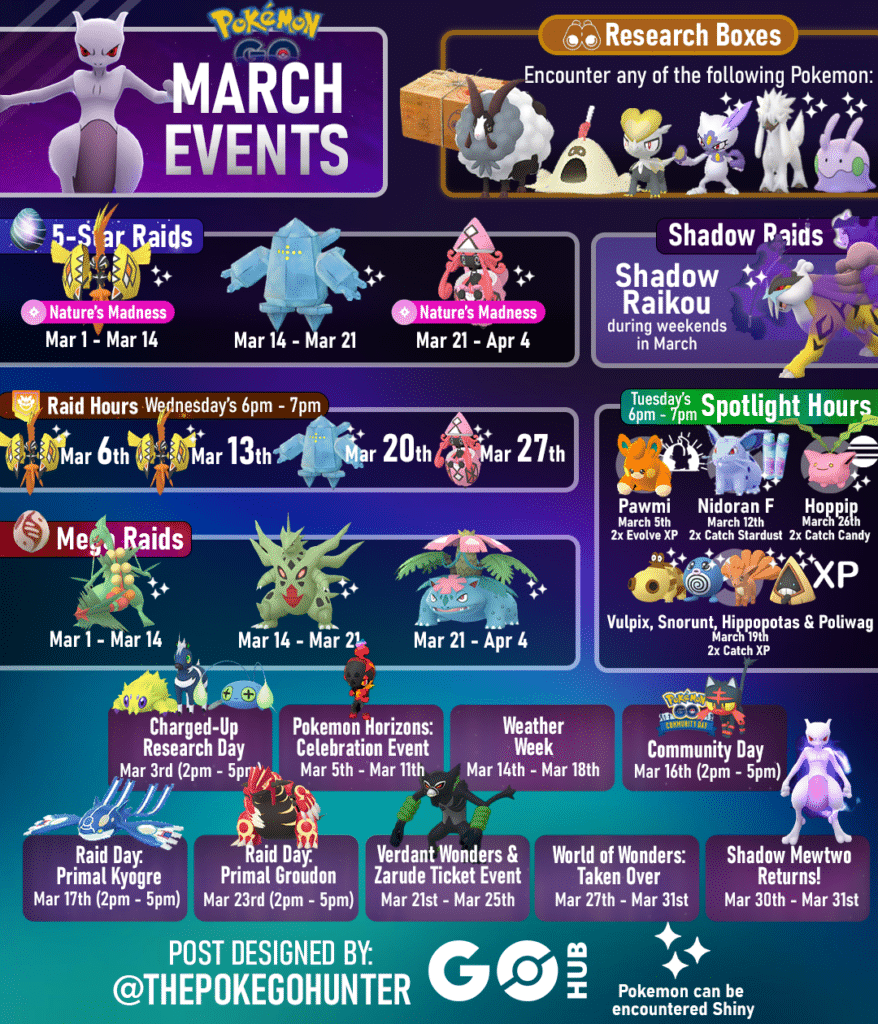The image features a gradient background transitioning from turquoise at the bottom to purple at the top. The main heading reads "Pokémon March Events." Below this, there is information about various in-game activities:

- **Research Boxes:** Players can encounter any of the listed Pokémon.
- **Five Star Raids:** "Nature Madness" will occur from March 1st to March 14th and again from March 21st to April 4th.
- **Shadow Raids:** Shadow Raikou will be available during weekends in March.
- **Raid Hours:** Scheduled every Wednesday from 6 PM to 7 PM on the following dates - March 6th, March 13th, March 20th, and March 27th.
- **Spotlight Hours:** Held each Tuesday from 6 PM to 7 PM, featuring:
  - March 5th: Palmy with 2x Evolve XP
  - March 12th: Nidoran♀ with 2x Catch Stardust
  - March 26th: Hoppip with 2x Catch Candy

Additional Spotlight Pokémon include Vulpix, Snorunt, Hippopotas, and Poliwag.